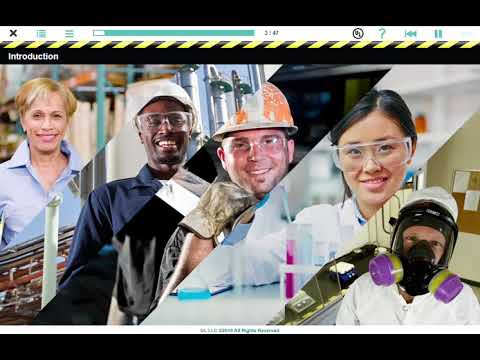The image shows five different faces of people presumably at their respective workplaces, set against a control bar indicative of a video playback interface. At the top, a thin blue playback bar stretches across the image, with an assortment of control buttons, including a black 'X' on the far left, two green dropdown menus next to it, and various other icons on the right, such as a question mark, a rewind button, and a pause button. Below this bar, "Introduction" is prominently displayed, flanked by warning stripes resembling black and yellow traffic lights. 

The main image consists of five individuals from left to right, each presumably engaged in their work:

1. A woman with short blonde hair, smiling and wearing a blue shirt, positioned in what appears to be a factory setting with construction materials in the background.
2. Next, a black man smiles while donning a white safety hat, clear protective glasses, and a dark blue shirt, with blue and silver pipes visible behind him, suggesting a machinery or construction environment.
3. Following him, a man sports an orange safety helmet, gloves, clear protective glasses, and holds a steel bar, implying a construction or industrial work site.
4. To his right, an Asian woman in clear protective glasses is smiling while carefully pipetting into a test tube, dressed in a white lab coat, clearly situated in a scientific laboratory.
5. Finally, a man in a white outfit and purple-nosed gas mask gazes intently at the viewer, surrounded by laboratory equipment and test tubes.

This detailed scene captures diverse professionals in their respective environments, illustrating various industrial and scientific fields.